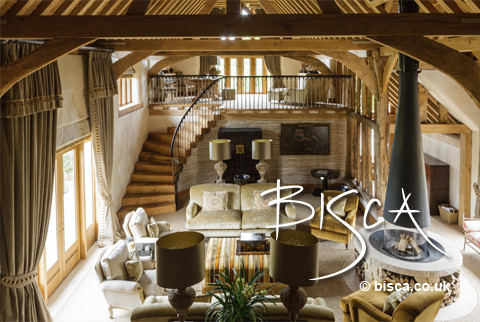This photograph captures the sophisticated, contemporary interior of a designer home, taken from an elevated viewpoint, possibly from a balcony or the rafters, looking down upon a spacious, open-plan living area. The home features a two-story layout with intricate wooden architectural elements, including rafters, joists, and angles that support the ceiling and extend to a second-floor loft area with a railing. Dominating the main floor is an arrangement of cushy, light-colored furniture, including a sofa and multiple chairs surrounding a wooden coffee table in neutral tones. A notable feature within the room is an open-air fireplace with a circular base, encased in glass, and a slim metal chimney stretching upward. Flanking the fireplace is a charming brick wall with wooden supports. The left side of the room exhibits very tall brown drapes next to a large doorway with glass panes, possibly leading outside. Curved, pottery-inspired lamps with tall, cylindrical brown shades provide ambient lighting. The space is elegantly designed, featuring additional details like a painting near a wooden staircase that ascends to the second floor. Soft sunlight filters into the room, giving a warm yet airy feel, and the overall upscale ambiance is accentuated by the curated mix of contemporary and rustic elements. At the bottom right of the image, a text overlay reads, "BISCA" with a stylized 'S', accompanied by "bisca.co.uk."